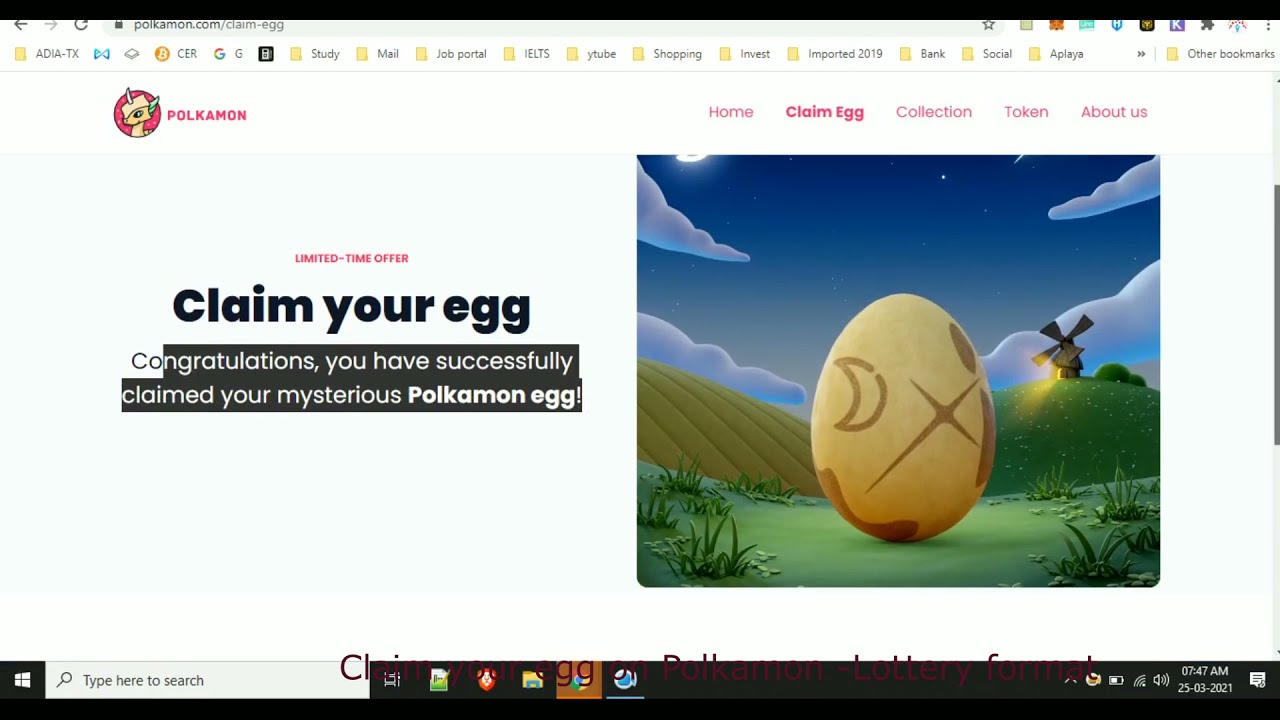This is a detailed caption for an image:

"A screenshot of a web page centered on a promotional section. On the left, in smaller red letters, it reads 'Limited Time Offer,' and in bold black letters below, 'Claim Your Egg.' Beneath this, it announces, 'Congratulations! You have successfully claimed your mysterious Pokémon egg.' To the right of this text is an image depicting a scene with a dark blue sky, scattered clouds, and rolling green hills in the background. In the foreground, a large yellow egg, adorned with a moon, a cross, and several dark brown patches, sits on the grass. The background also features a windmill emitting a yellow light and surrounded by green plants. Above the promotional section, the page header displays 'Pokémon,' with navigation options labeled 'Home,' 'Claim Egg,' 'Collection,' 'Token,' and 'About Us.' The bottom of the page is marked by a black banner containing a search bar and various icons."